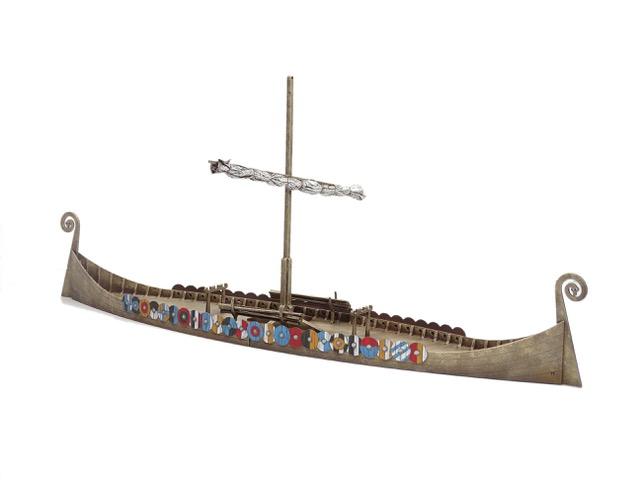This detailed drawing features a Viking-like ship rendered against a minimalist white background, implying an outdoor setting. The ship, likely a model, prominently features an ornate single mast with the sail tied up and an arm crossing the mast. The mast itself is visually striking, ending in decorative elements that curve and swirl upwards, likely resembling snake heads. Both ends of the boat mirror these elegant swirling designs. 

The ship's deck appears broad, with meticulously detailed support beams lining the cutouts along either side. Perhaps the most vibrant aspect of the drawing is the array of circular lifesavers—described as wooden circles or album-like wheels—that adorn the ship's edges. These lifesavers come in a myriad of colors and patterns, including solid reds, browns, blues, and blacks, along with striped combinations like blue-and-white, black-and-white, red-and-brown, and various other mixtures. Each side of the ship features approximately 20 of these colorful discs, each adding a unique burst of color to the intricate vessel. Notably, the boat is devoid of any people or text, allowing the focus to remain solely on the ship's detailed craftsmanship and vivid embellishments.